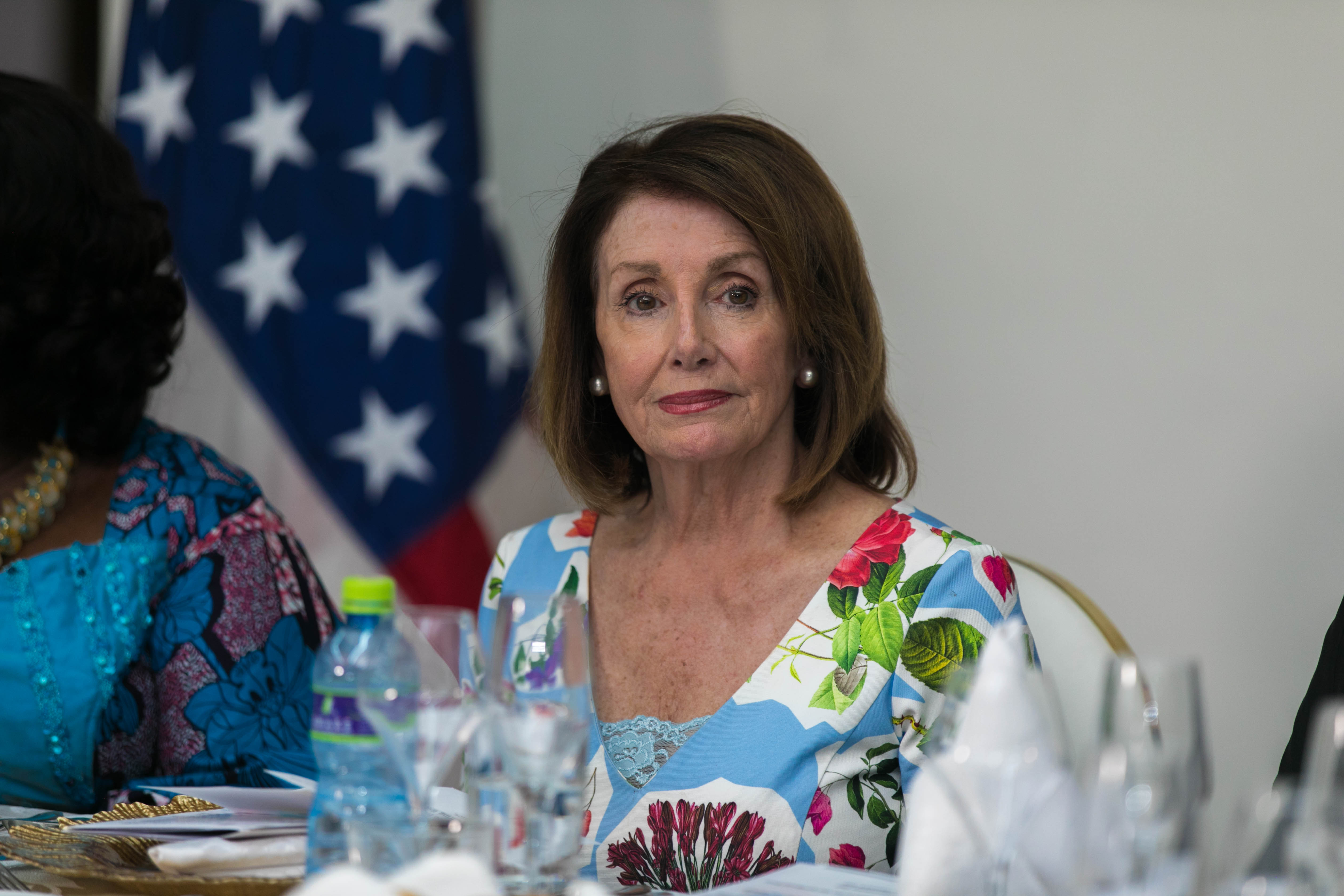The photograph features an elderly white woman, identified as Nancy Pelosi, seated at a table. Nancy, who appears to be in her 80s, has short, shoulder-length brown hair and is wearing striking, large, silver-colored pearl earrings. She is dressed in a multicolored floral blouse or dress, predominantly blue and white, adorned with red roses, purple flowers, and green leaves. The dress has a V-neck neckline embellished with a piece of lace at the center. The table in front of her is cluttered with various objects, including bottled waters, plates, glasses, trays, and pamphlets. An American flag is positioned prominently in the background against a white wall. Also visible in the photograph is another elderly woman with short black hair, dressed in a blue dress. The setting appears to be indoors, likely within a government building, given the formal arrangement and presence of the flag. The overall image displays a range of colors including blue, red, green, purple, and gold.